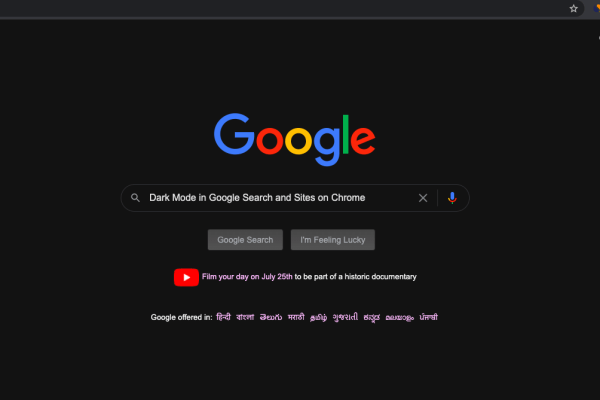A detailed caption for the image described:

"This color landscape screenshot captures the classic Google web browser interface in dark mode. The familiar Google logo is prominently displayed against a sleek black background; it features a blue capital 'G', followed by lowercase letters 'o' in red, 'o' in yellow, 'g' in blue, 'l' in green, and 'e' in red, with the 'e' tilted slightly upward. Within the search bar, the text reads 'dark mode in Google search and sites on Chrome,' indicating a user preference likely geared towards more comfortable nighttime browsing.

Below the search bar, the options for 'Google Search' and 'I'm Feeling Lucky' are available, offering users the choice between receiving a full list of search results or being taken directly to the top search result. Beneath these options, there is an announcement featuring the YouTube logo and an invitation to 'film your day on July 25 to be part of a historic documentary.' Additionally, a note at the bottom highlights that Google is offered in multiple languages, each one listed as a translated alternative."